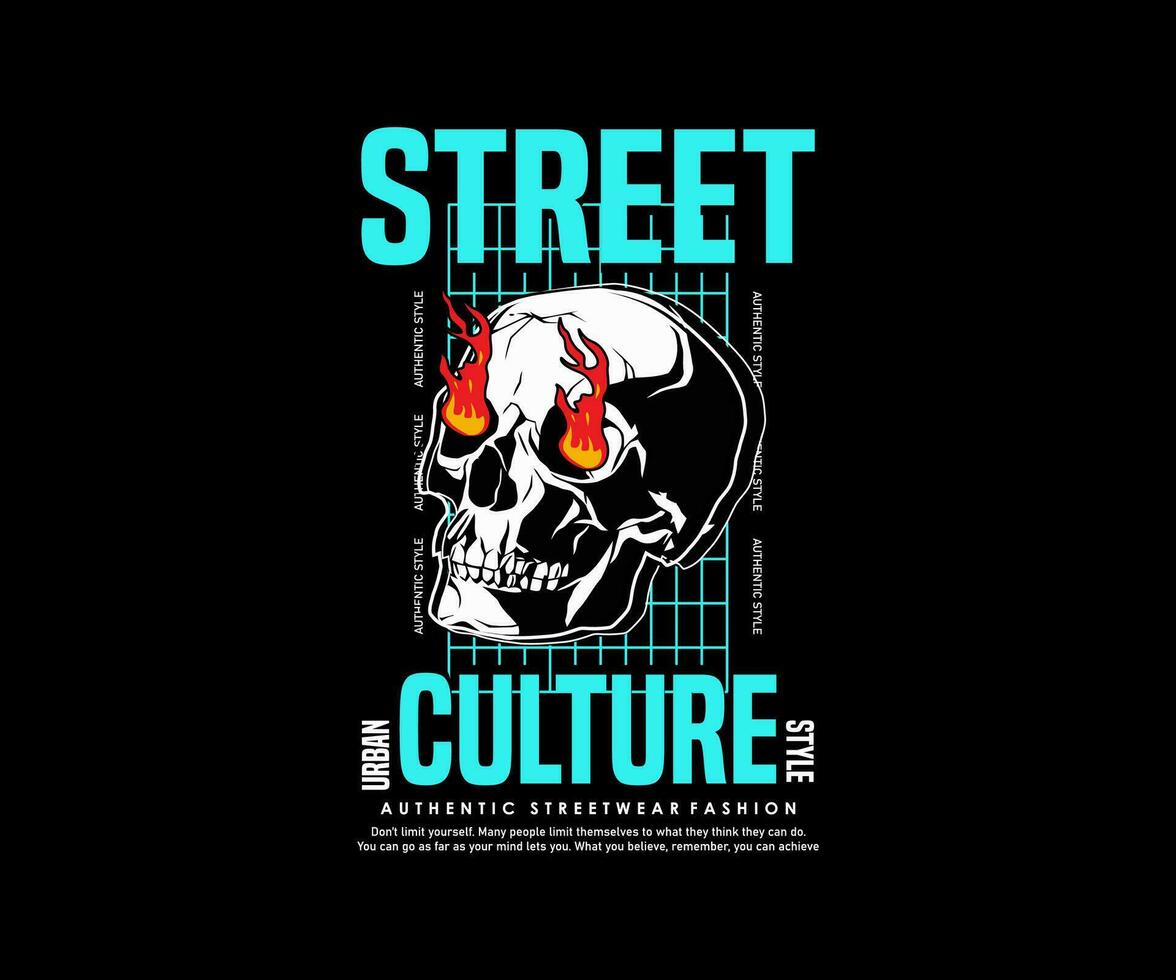This graphic, which appears as though it could adorn a t-shirt, is set against a solid black background. Positioned centrally within a large black square, the top of the design features the word "STREET" in striking cyan capital letters. Dominating the middle of the composition is a complex black and white skull, vividly detailed with intricate cracks and teeth, embellished with vector-styled flames erupting symmetrically from its eye sockets; the flames transition from yellow at their base to red at their tips. Behind the skull, a subtle cyan grid pattern adds a layer of dimension. The word "CULTURE" echoes in large cyan capitals at the bottom of the graphic. Flanking this are the words "URBAN" on the left and "STYLE" on the right, both in white vertical uppercase letters. Beneath "CULTURE" is a smaller text block that reads "AUTHENTIC STREETWEAR FASHION," alongside an inspirational message: "Don't limit yourself. Many people limit themselves to what they think they can do. You can go as far as your mind lets you. What you believe, remember, you can achieve."